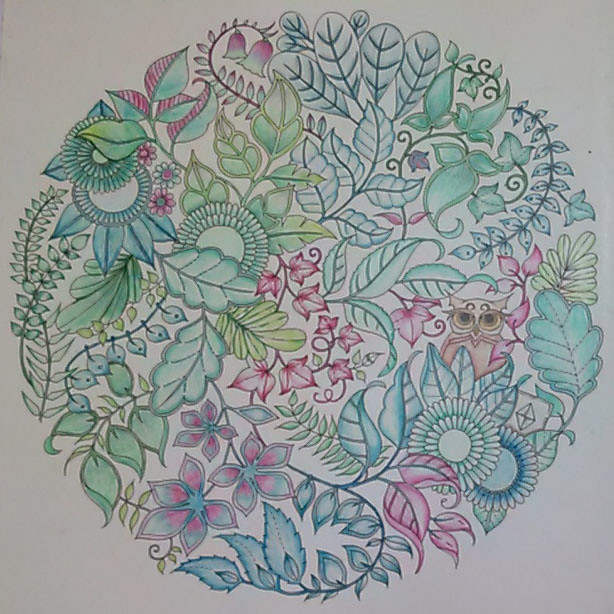This real-life photo captures a meticulously illustrated design on a pristine white piece of paper. Dominating the composition is a circular arrangement, crafted from an intricate tapestry of various plant elements. These plants manifest in a harmonious blend of hues—bright green, dark blue-green, teal, and sea green—complemented by delicate touches of pink. The illustration is reminiscent of a floral pattern, featuring an array of intertwining vines, diverse leaves, and flowers that intriguingly mimic foliage. Each element interlocks with the next, forming a graceful, interconnected circle.

Amidst this verdant assembly, a cleverly concealed owl peers out, its presence discernible by its large, expressive black eyes and brown plumage, subtly obscured by surrounding leaves. The composition features numerous swirling tendrils and elegantly curling leaves, enhancing the dynamic interplay of shape and color. The contrasting shades of blues and greens contribute depth and texture, creating a captivating visual experience that invites closer inspection to uncover its hidden intricacies.